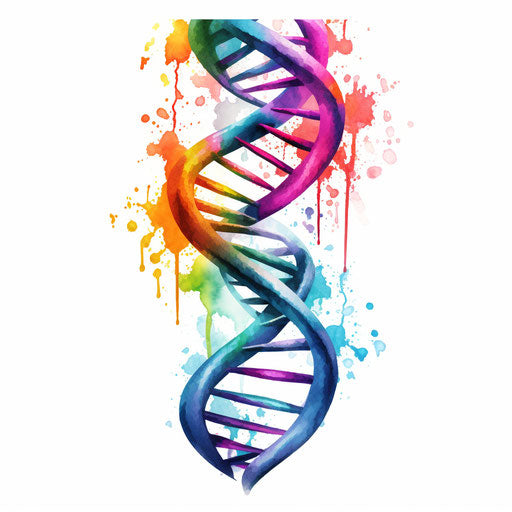This image is an art piece depicting a double helix DNA strand, skillfully rendered in watercolor. Taking a central position on the canvas, the DNA strand resembles a gracefully twisted ribbon, evoking the structure of a flexible ladder spiraling upwards like a staircase. The vibrant color gradient begins with blues and purples at the base, transitioning through deeper shades of purples to greens, and culminating in warm hues of oranges and reds towards the top. Additionally, the colors bleed into the background, creating splotchy splatters: reds and pinks correlate with the red and pink sections of the helix, oranges with oranges, and greens and blues respectively splatting into their corresponding hues. These splatters add to the overall dynamic and somewhat cartoony aesthetic, all set against a stark white backdrop, enhancing the vividness of the colors. Overall, the artwork becomes more colorful and visually arresting as the eye moves upward, imbuing the piece with a lively and dynamic feel.